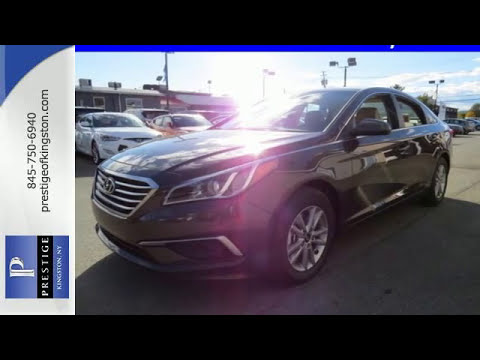The image features a modern, sparkling purple Hyundai sedan parked in a sunlit car lot. The intense sunlight reflects off the car's hood and bumper, creating bright, overexposed highlights. To the left of the car, several other vehicles are visible, along with what appears to be an apartment complex in the background. On the right side of the image, a vertically oriented business sign displays the name "Prestige" along with a logo, a phone number (845-750-6940), and the website "prestigeofkingston.com," indicating that the car is likely for sale through Prestige of Kingston, NY.